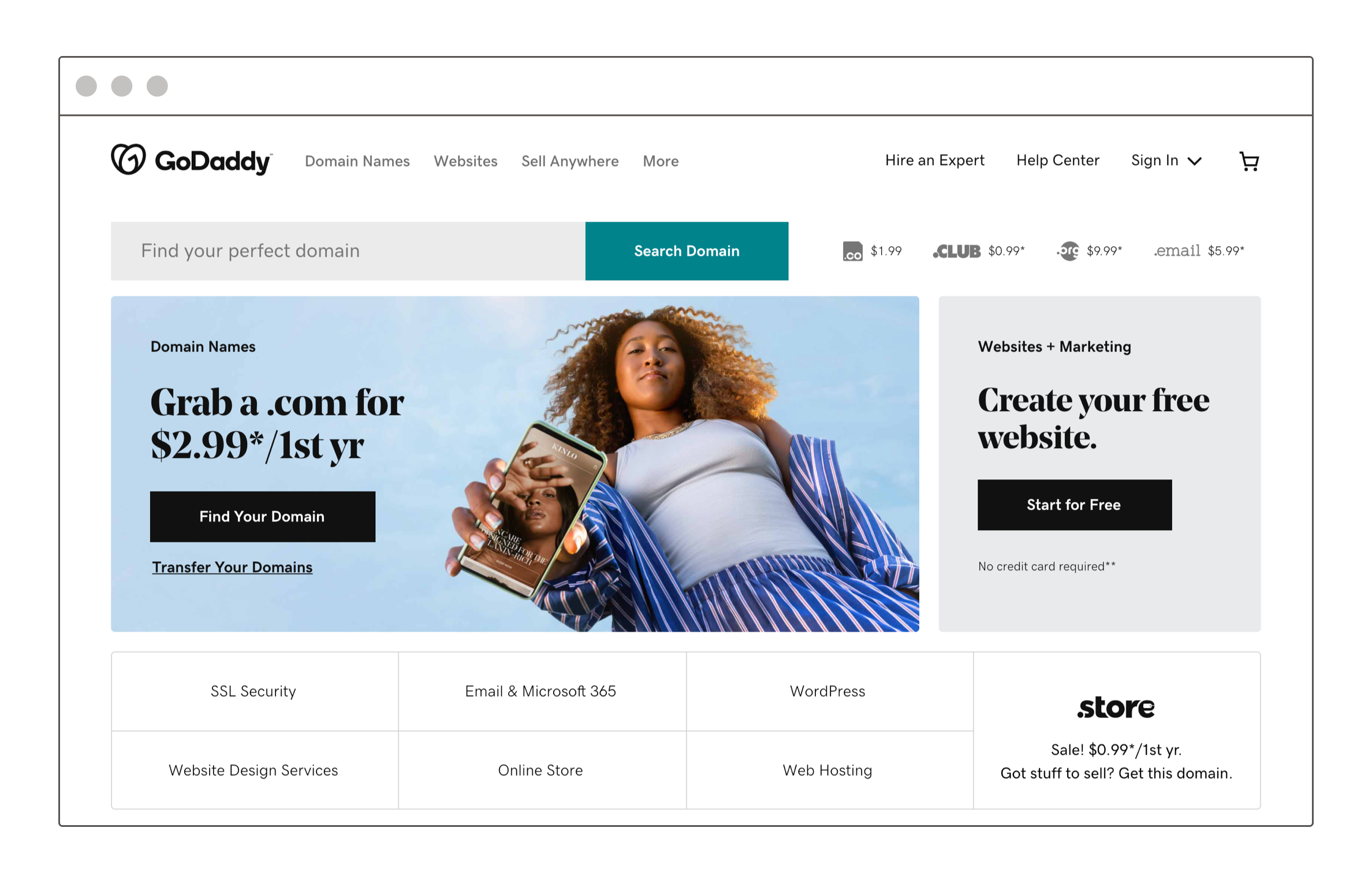This is a detailed screenshot from GoDaddy.com, a popular website creation and domain registration service. The top navigation bar includes options such as "Domain Names," "Websites," "Sell Anywhere," and more. On the right side, users can access "Hire an Expert," "Help Center," and "Sign In." A prominent search bar invites users to "Find your perfect domain," accompanied by a search function and a tilde button.

A large advertisement prominently displays an offer for .com domain names at $2.99 for the first year, highlighted by a star symbol. The ad encourages users to find their domain and also offers a link for domain transfers.

The focal point of the image is a photo of tennis star Naomi Osaka, who is depicted looking down against a backdrop of clear sky. She is dressed in a gray tank top paired with a white and blue plaid shirt and pants, and she holds a cell phone downward. This image appears to be linked to her website.

The page features a section titled "Websites + Marketing," which promotes the creation of a free website with no credit card required to start. Below this, several other site options are presented, including SSL Security, Email & Microsoft 365, WordPress, Website Design Services, Online Store, and Web Hosting. A special offer is highlighted for .store domains at $0.99 for the first year, suggesting this as an ideal solution for those with items to sell.